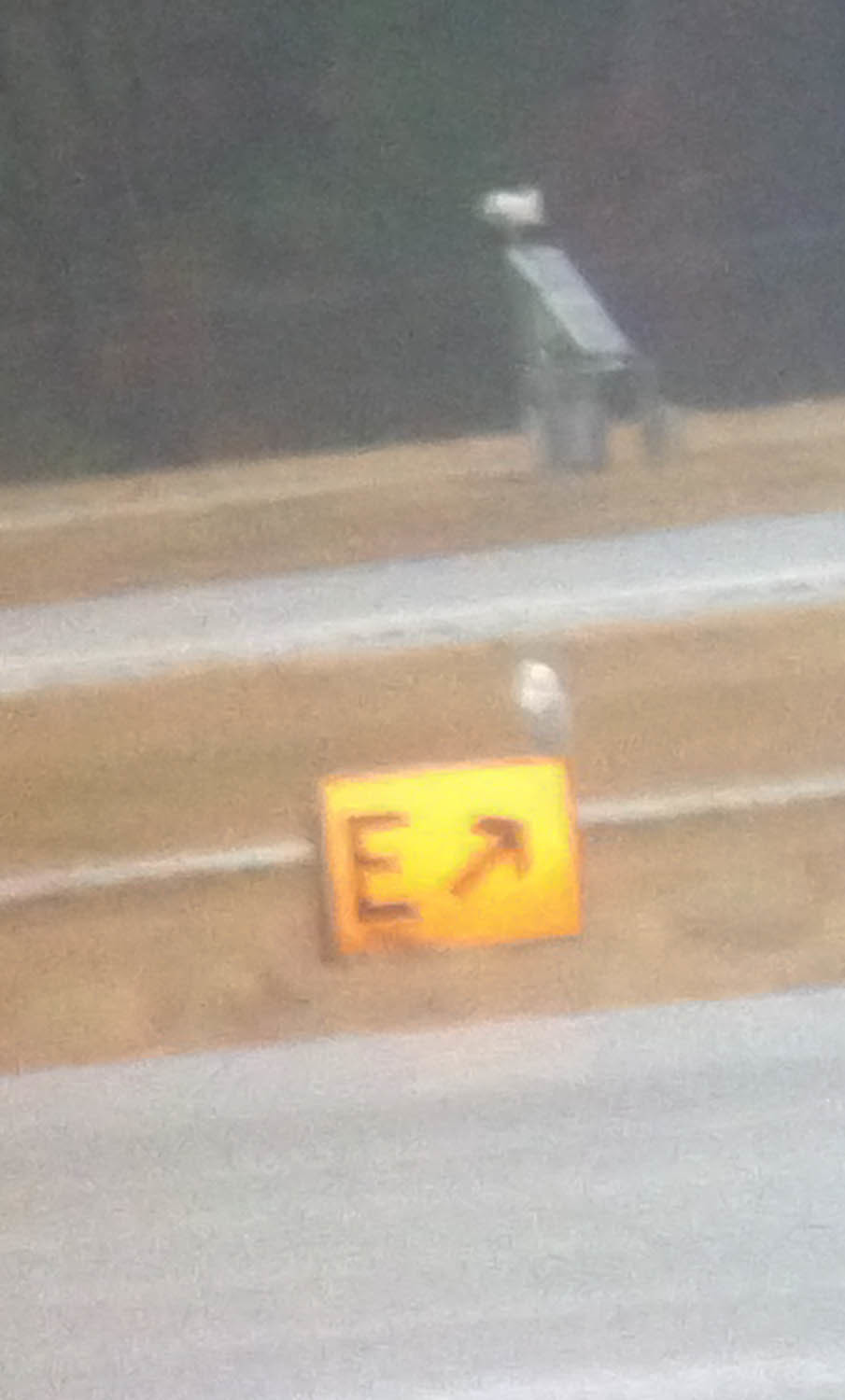The image is a blurry, first-person POV photograph, vertically oriented and appearing to be taken in motion, likely from a vehicle on a road. The foreground shows a gray road covering the bottom fifth of the image. Above the road, a brown, wooden wall occupies the midsection of the background, housing a prominent yellow sign. This sign features a black letter "E" and a black arrow pointing diagonally upwards to the right. Positioned behind the yellow sign is a silver or white pole. Slightly to the right and above the center of the image, there's a mechanical object resembling a silver faucet or sink fixture. The far background showcases alternating strips of grass and road, with tree lines in the distance, and the top portion of the image fading into blackness.